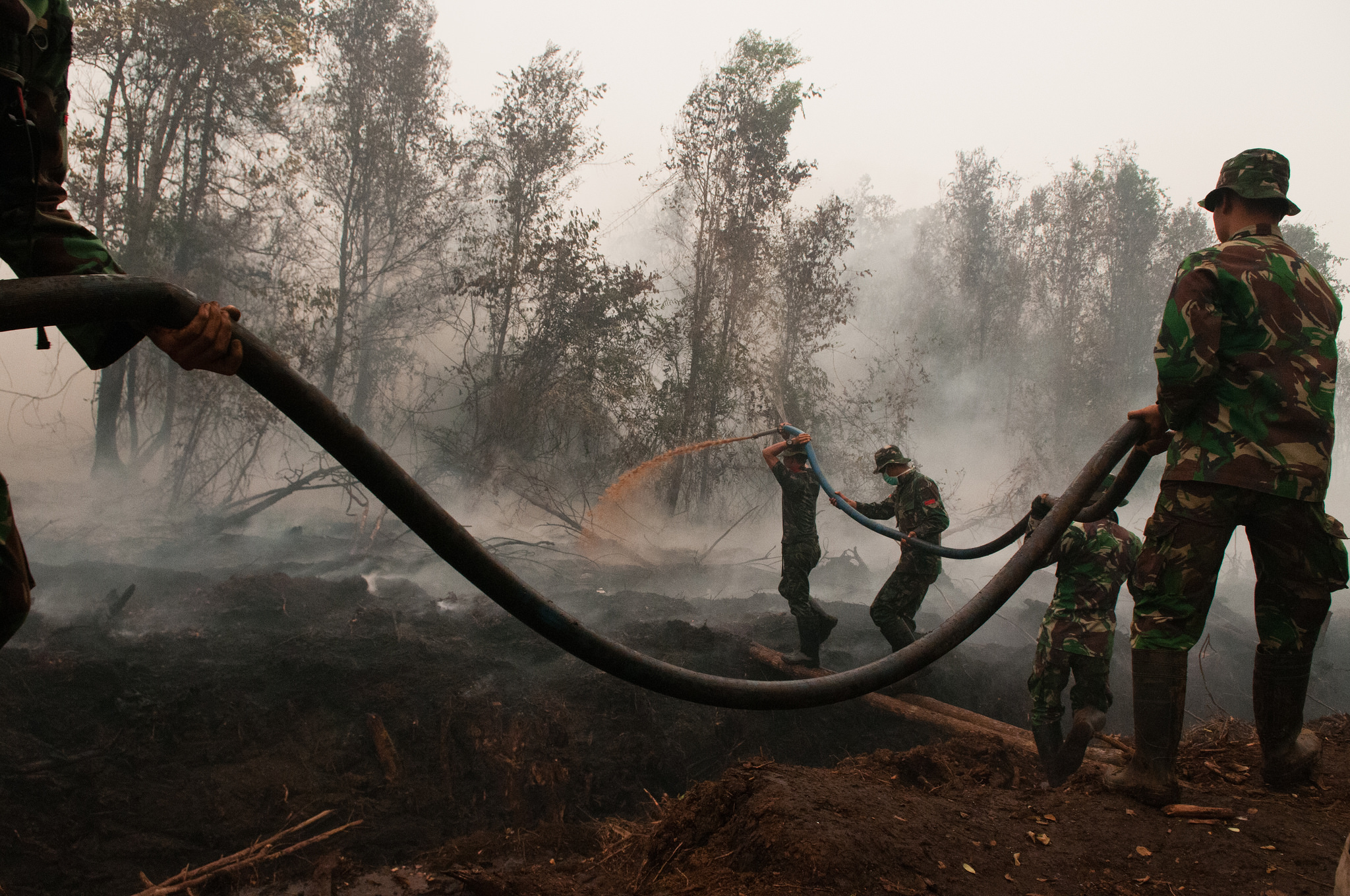In the aftermath of a forest fire, a group of five military members clad in camouflage uniforms are seen battling the lingering flames. Amidst a charred and smoldering landscape, where the ground is blackened and strewn with fallen trees, they diligently aim a fire hose spewing brownish water onto the smoking remnants. The air is thick with white smoke, partially obscuring the tall trees in the background. One of the soldiers, distinguished by his camo-patterned boonie hat, is positioned to direct the water, while the others support the hose, guiding it along its length. The scene is cloaked in an eerie fog, with the sky completely overcast by the dense smoke, rendering the devastation of the blaze palpable.